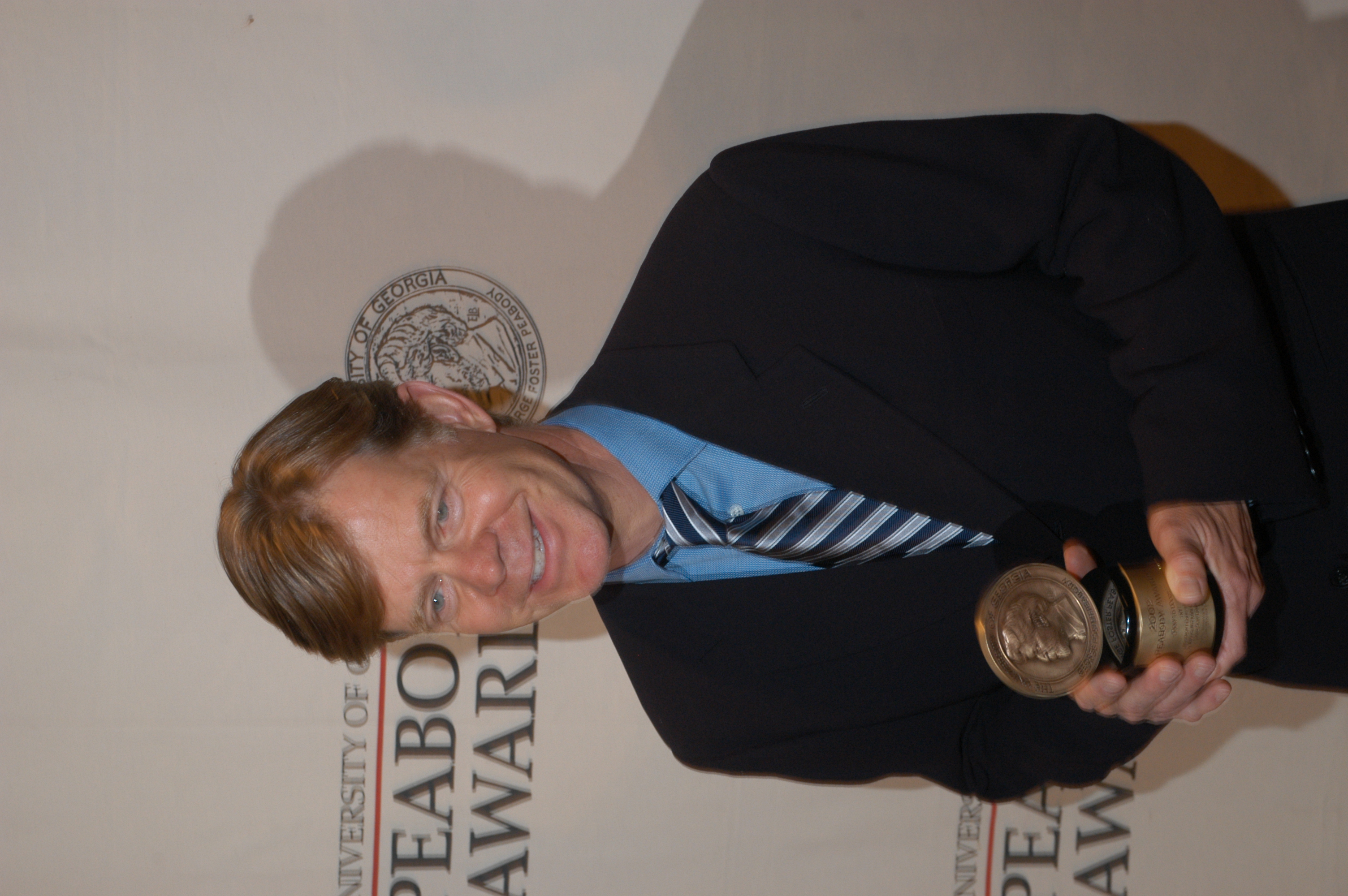The photograph features a middle-aged white man, possibly in his 50s or 60s, who bears a resemblance to William H. Macy. The image is slightly rotated, positioning the man's head towards the left and his legs towards the right. He is depicted from the waist upwards, dressed in a formal black business coat over a blue button-up shirt with prominent white buttons, and a gray and black striped tie. In his hands, he holds a large, round coin trophy mounted on a cylindrical base, which displays a side profile of a man, evoking a Greek-themed design. The background consists of a white wall emblazoned with part of a banner that reads "University of [cut off] Peabody Awards" in black text alongside a graphic that mirrors the coin trophy he is holding.